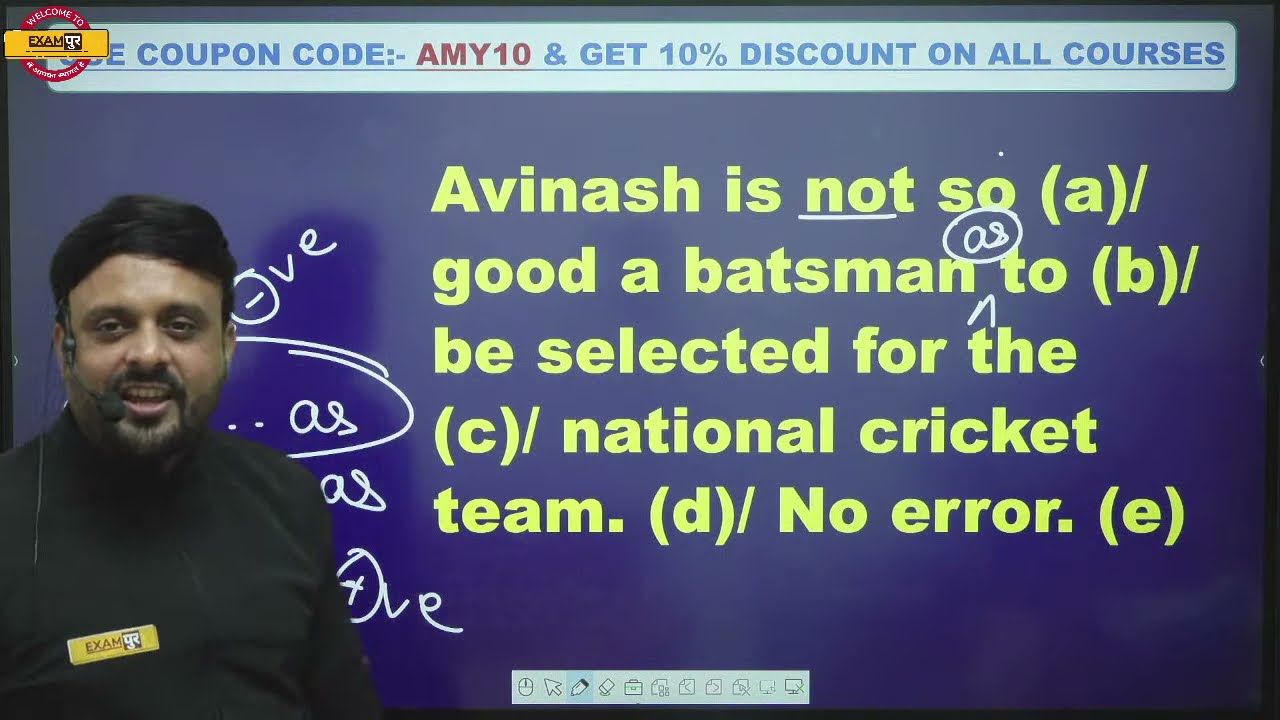In the image, we see an Indian man standing on the left side, wearing an all-black outfit with a rectangular badge on his chest that reads "Exam." He has black hair, neatly combed to the side, and a light black beard and mustache. The man is equipped with a microphone attached to an earpiece, suggesting he's delivering a lecture or presentation. Behind him is a large dark blue screen with several texts displayed. At the very top, in light blue and red text, it reads, "Use coupon code AMY10 and get 10% discount on all courses." Below this, in yellow text, it says, "Avinash is not so good a batsman to be selected for the national cricket team. No error." The screen and the context imply that this is an educational course, possibly focused on English language lessons, where the man appears to be explaining or discussing content. Additionally, on the top left corner, there is an orange banner with the word "Exam" and a symbol beside it, with a red ring and unreadable white text behind it.